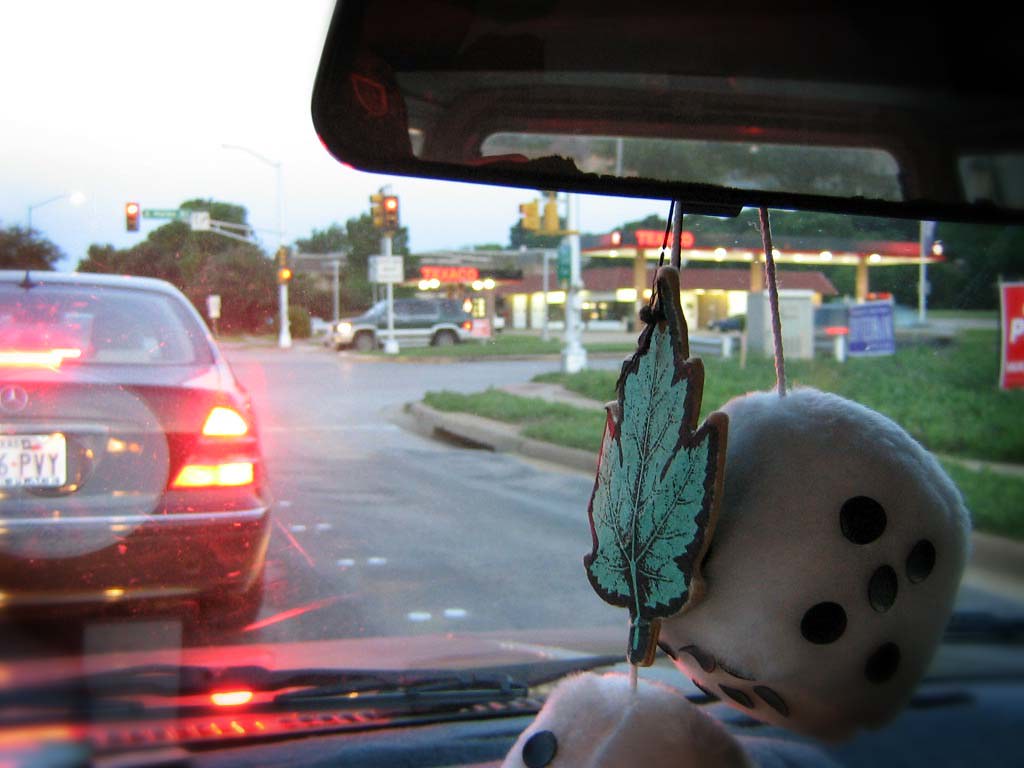This is a vivid color photograph taken from within a vehicle, capturing a blend of interior and exterior details. Prominently at the top right of the image is the car's rearview mirror, which hangs an assortment of items: a green, leaf-shaped air freshener and a pair of white fuzzy dice. Through the windshield, the view ahead reveals a dark-colored Mercedes with its brake lights and tail lights activated. The vehicle's partially visible white license plate prominently displays the letters "P-V-Y." In the background, traffic lights glow red, indicating a stop, and to the right of the scene, a Texaco gas station punctuates the urban setting, while a patch of green lawn adds a touch of nature. Notably, there are no people present in the photograph, enhancing the focus on the serene yet detailed cityscape and the array of elements inside the vehicle.